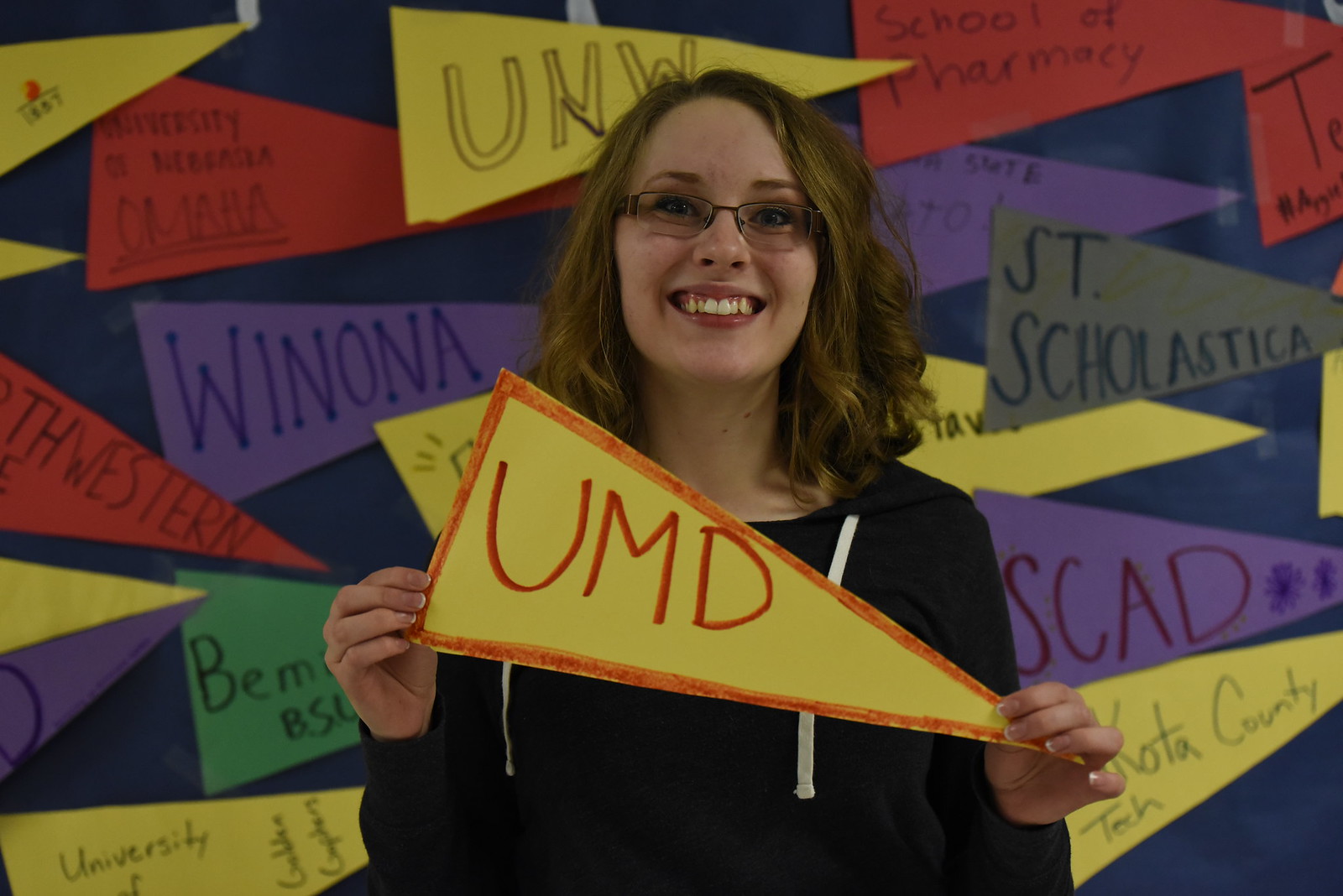In this image, a young Caucasian woman with shoulder-length curly brown hair and prescription glasses is smiling brightly, showing her teeth and even her eyes seem to be smiling. She is wearing a black hoodie with white drawstrings and holding up a handmade, triangular yellow banner that has a red border and red letters spelling "UMD." The background features a blue wall adorned with similarly shaped and colorful cardboard cutouts with the names of various universities and colleges displayed. These banners come in a variety of colors including red, yellow, purple, green, blue, and gray. Some of the visible names on these banners include SCAD, St. Scholastica, School of Pharmacy, UNW, Winona, and University of Nebraska Omaha, adding a diverse and vibrant academic theme to the scene.